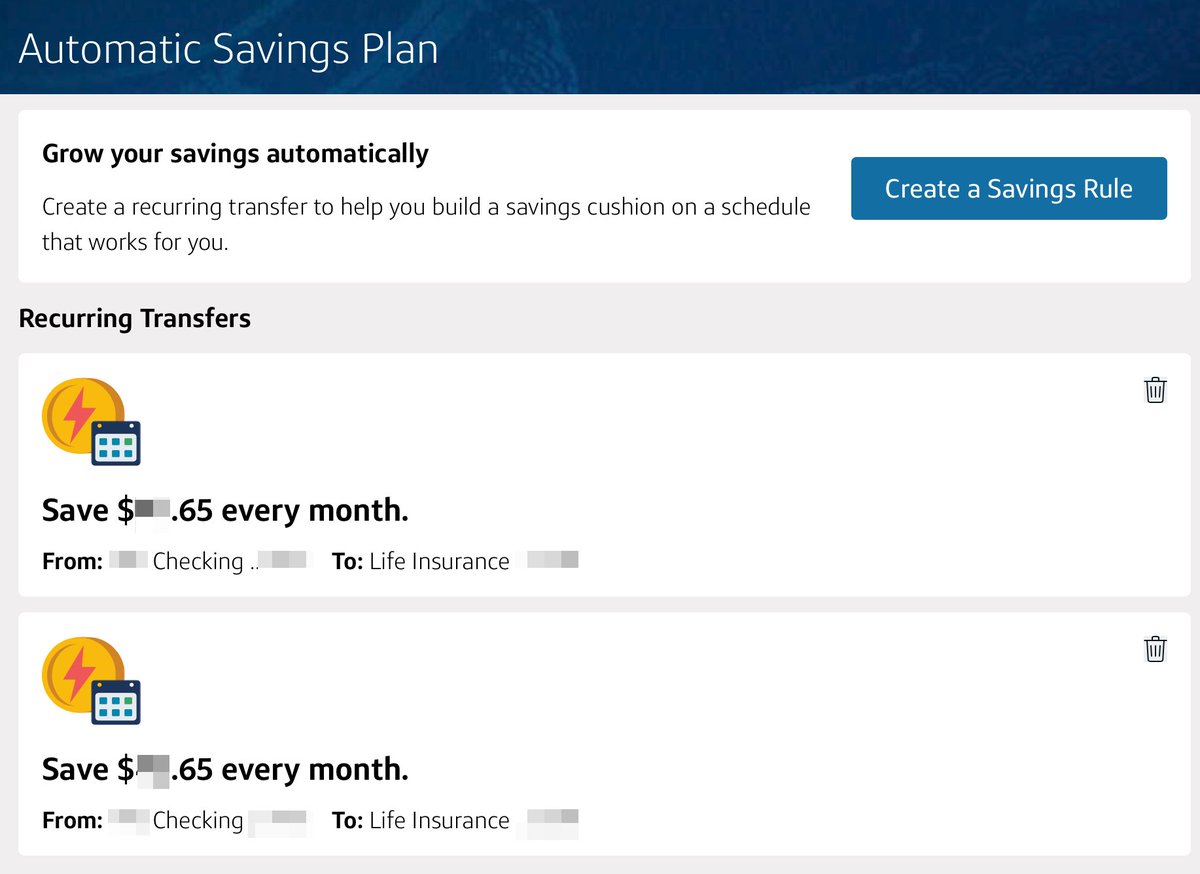This screenshot is from the background of an app or website focused on savings accounts and savings information. At the top, a long blue rectangular banner prominently displays the text "Automatic Savings Plan" in white. Beneath this banner, there are three distinct white rectangular boxes.

The first white box features the heading "Grow Your Savings Automatically" in bold black text. Below this heading, it provides the description: "Create a recurring transfer to help you build a savings cushion on a schedule that works for you." On the right side of this box, there's a lighter blue rectangular button labeled "Create a Savings Rule." Underneath the main text, this section is also marked with the term "Recurring Transfers."

In the second white box, there's a small yellow icon next to the text "Save $0.65 every month from checking to life insurance," accompanied by a trash icon located on the right side of the box, indicating options for deletion or modification.

The third white box mirrors the second, repeating the text "Save $0.65 every month from checking to life insurance," along with another trash icon on the right. Each of these white boxes also includes a small yellow icon with a red lightning bolt inside, as well as two smaller boxes containing multiple green and blue squares, providing additional visual details related to the savings rules and their functionalities.